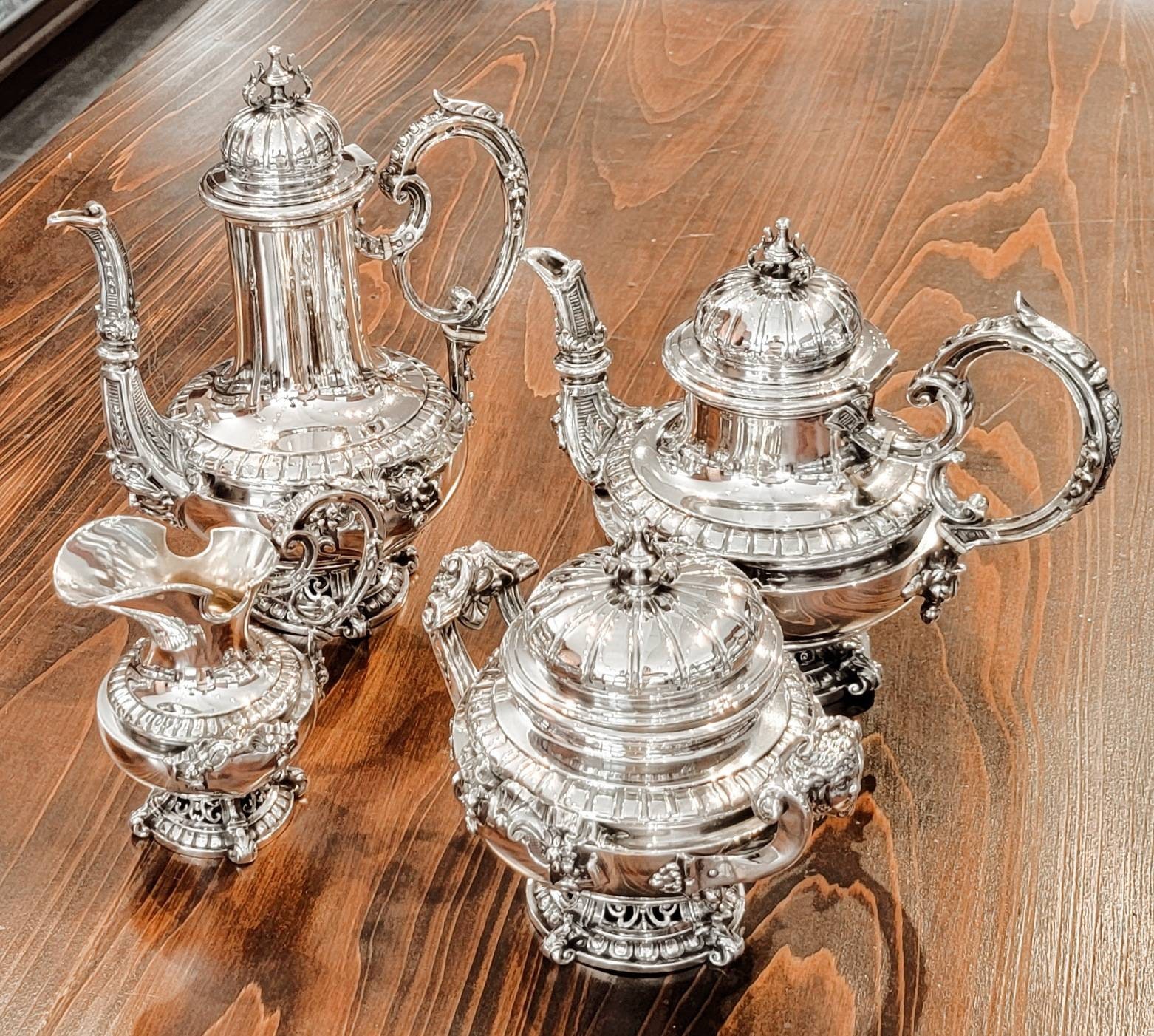This detailed color photograph showcases an antique silver tea and coffee set, elegantly arranged on a dark walnut-colored wooden table with visible wood grain patterns. The set includes four highly polished, ornate pieces. In the back, there's a tall tea pitcher with a long spout and capped top, accompanied by a slightly shorter coffee pitcher with similar features. Both pitchers are beautifully crafted with large, ornate handles. In front of the tea pitcher, there is a smaller open cream or milk jug, featuring a curved spout and an equally ornate handle. Situated beside the jug, in front of the coffee pitcher, is a roundish sugar bowl designed for holding sugar cubes. The harmonious arrangement of these antique silver pieces against the rich wooden surface creates a striking visual contrast, with the dark outer rim of the table adding a touch of sophistication to the scene.